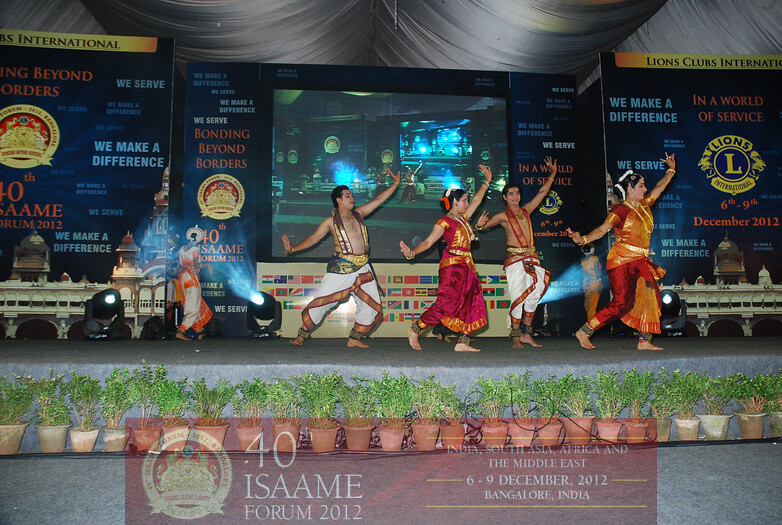The image is a horizontally oriented photograph capturing a performance on a narrow concrete stage during the 40th ISAAME Forum held in Bangalore, India, from December 6th to 9th, 2012. Four dancers clad in traditional Indian attire—comprising long, flowy pants and headpieces with colors including white, orange, and red—are performing an ethnic dance, holding dynamic poses with their hands in the air. Behind them, large blue placards tower approximately 20 feet high, with the one on the right declaring "Lions Club International," and the central and left ones displaying the event theme, "Bonding Beyond Borders" as well as the slogan "We Make a Difference." Additionally, the central placard features a live video stream of the dancers' performance. Striking curtain-like decorations descend from the ceiling on the stage, adding to the festive ambiance. A multitude of potted green plants adorn the foreground, just in front of the stage, and a lower sidewalk bordered by a "40 ISAAME" banner completes the scene. Bright lighting enhances the vividness of the dancers' movements, reflecting the celebratory spirit of the event.